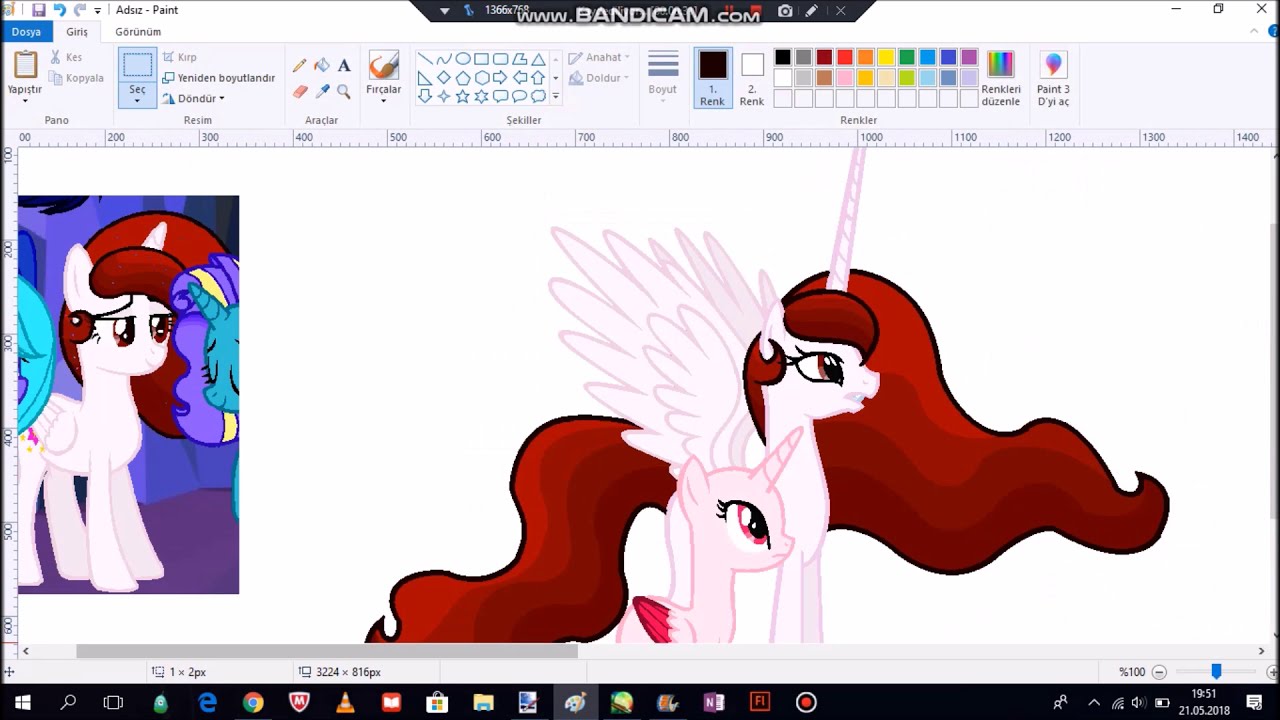This is a horizontal rectangular screenshot from a computer displaying an Adobe Paint workspace. At the very top, it reads "Adobe Paint," and just below that, across the center, is the text "www.bandicam.com." The main canvas shows a white background featuring two unicorn drawings. The central focus is a large white unicorn with a tall horn, pegasus wings, and long, wavy red hair, flowing gracefully in both directions. Adjacent to her is a smaller pink unicorn, visible only by its head and neck, which lacks a mane but also has a horn. To the left within a purple rectangular clip, there's a detailed image of a white unicorn with long, wavy red hair, though it is unclear if it's the same unicorn depicted on the central canvas. The right margin of the image is partially cut off, showing a blue unicorn with a mixture of yellow and purple mane. The interface includes visible editing tools for color palettes and shapes at the top, and icons for applications like Internet Explorer and McAfee are seen along the bottom of the screen.